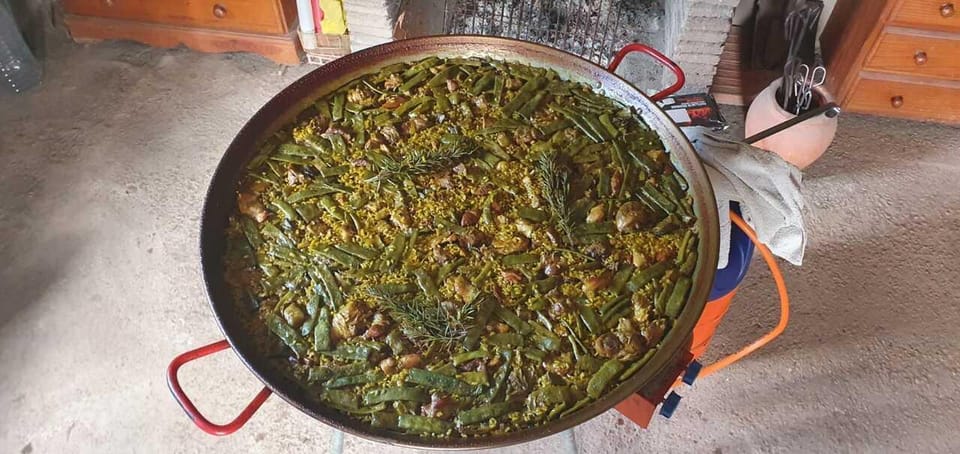The image is a landscape-oriented color photograph showcasing a large, shallow, round cooking vessel resembling a giant wok, made of metal with a bronze hue. It features two curved red handles on opposite sides. The vessel is filled with a cooked dish, predominantly composed of green vegetables such as rosemary, green beans, and possibly broccoli or kale, interspersed with beige elements like mushrooms, all immersed in a gold-colored sauce. There are also hints of brown, likely some variety of beans. The wok sits on a gray stone or concrete floor, indicative of a kitchen setting. Adjacent to the pot on the right is an orange-colored item with a string and a jar with scissors protruding from it. The background includes a light golden-colored wooden dresser on both the left and right sides and a brick fireplace with a partially visible grate in the center, enhancing the warm and rustic atmosphere of the room. The style of this photograph leans towards representational realism and is characteristic of food photography.